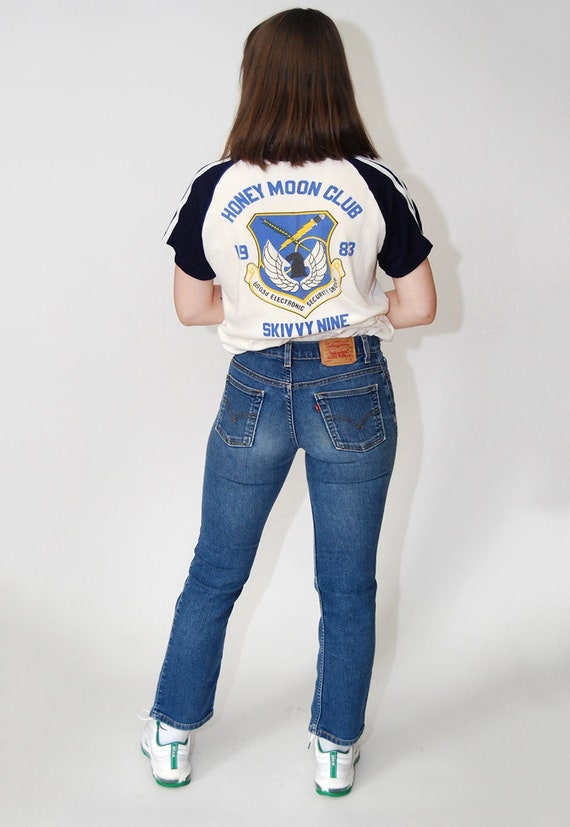A woman with straight shoulder-length brown hair is seen from behind, standing against a flat white backdrop that casts a faint shadow of her figure. She is dressed in a white t-shirt with black short sleeves, tucked into her jeans. The back of her shirt prominently displays the text "Honeymoon Club, 1983, Skivvy 9" above and below an emblem featuring a night chess piece surrounded by white wings, a lightning bolt, and a pole intersecting on a blue background. She completes her outfit with white tennis shoes accented by green. Her arms are bent at a 90-degree angle at her sides, and she is positioned to emphasize the details of her clothing and the shirt's graphic design.